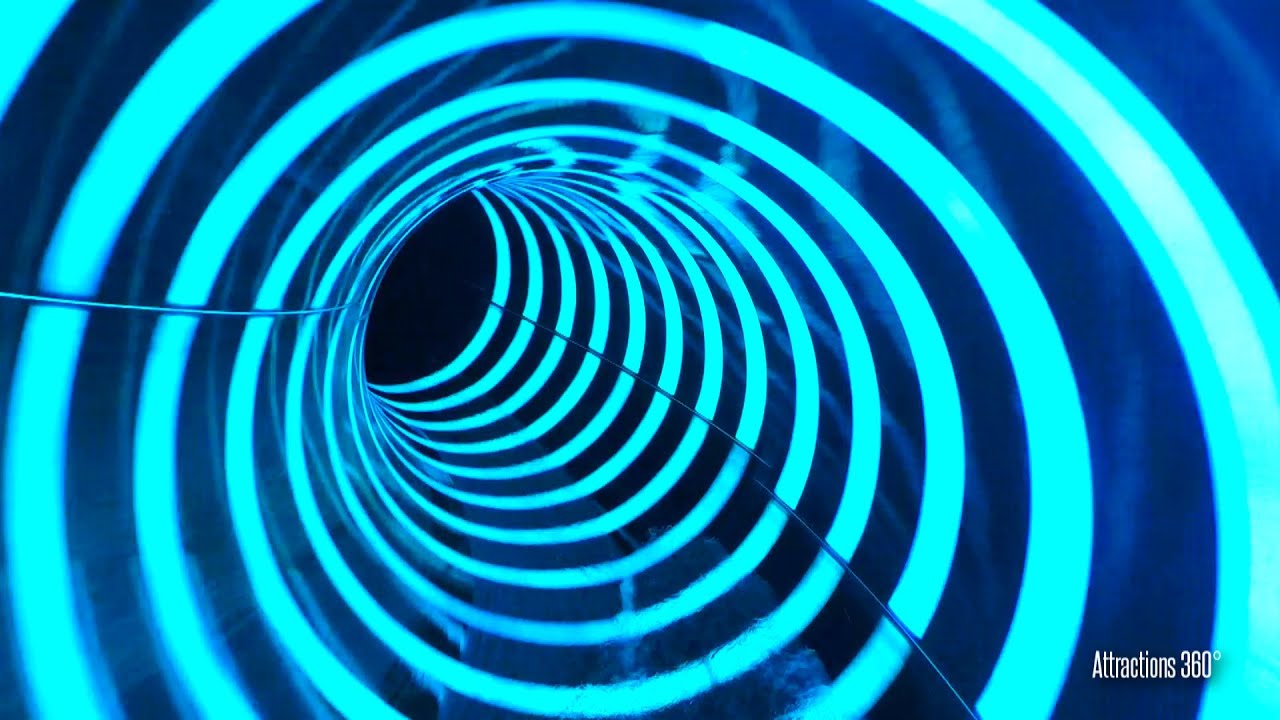The image is a color photograph labeled "Attractions 360" with a degree symbol in the bottom right corner. It depicts the interior of a large, enclosed dark blue tunnel, resembling a water slide. The tunnel curves to the left and extends into a black background. The inside of the tunnel is lined with bright aqua tube lights, creating a glowing, neon-like experience. These lights spiral in even intervals from the background to the foreground. Two black lines run parallel on both sides of the tunnel, possibly serving as wiring or bracing for the illuminated rings. Reflections of the lights are visible throughout the tunnel, enhancing the vibrant and immersive atmosphere.